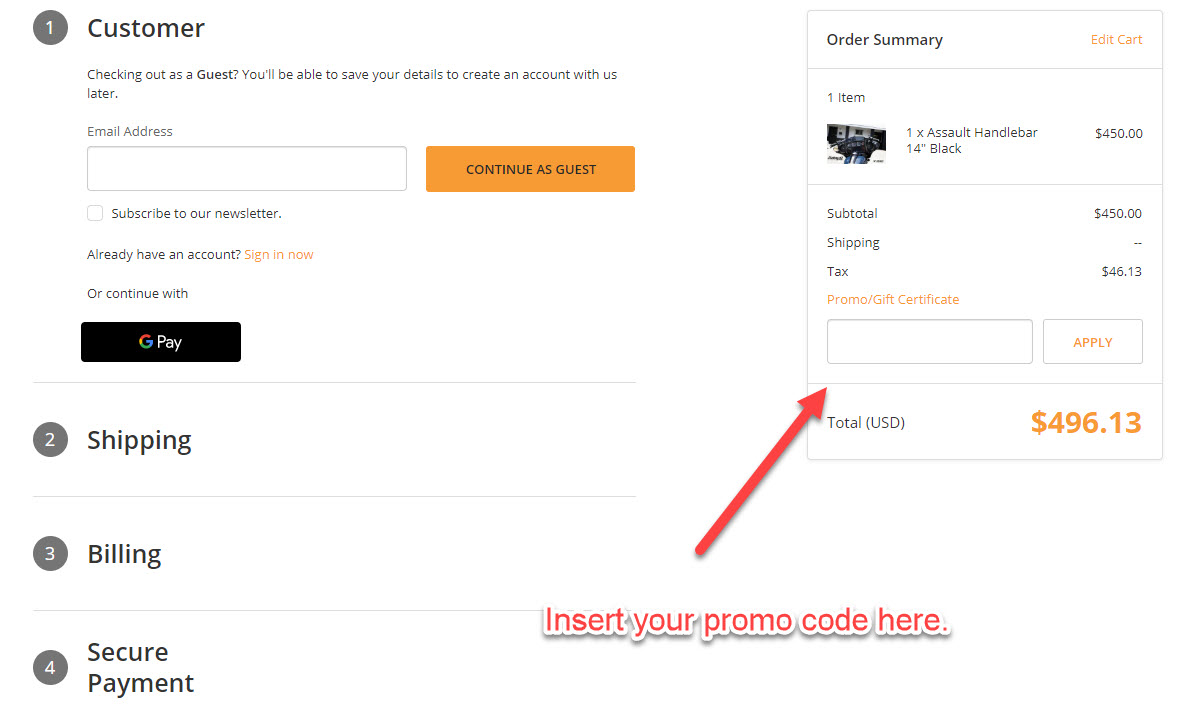**Image Description: Online Checkout Page**

The image depicts an online checkout page with a clean, white background. In the upper left corner, there's a gray circle with a white number "1" inside it, indicating the first step of the checkout process. Next to this, in black text, it reads "Customer" and underneath it says "Checking out as guest. You'll be able to save your details and create an account with us later." Below this text, there's a gray field labeled "Email," accompanied by a box where the user can enter their email address.

Beneath the email input field, there's an orange button with black text that says "Continue as Guest." Under this button, an option to subscribe to the newsletter is available, and there’s black text that reads, "Already have an account? Sign in now," next to an orange "Sign in now" button. Additional options include a "Continue with Google Pay" button.

Further down, there's a series of gray circles with white numbers "2", "3", and "4" inside them, labeled "Shipping," "Billing," and "Secure Payment," respectively, indicating the subsequent steps in the checkout process.

On the upper right-hand side of the page, there's a black bar with the text "Order Summary" in black. To the right, there's an "Add to Cart" button in orange. Below this, the order items are listed: "1x Assault Handle Bar, 14 inch, Black"—presumably for a motorcycle—priced at $450. The subtotal is listed as $450, with no additional cost for shipping. Tax is calculated at $46.13. There's a section for applying a promo or gift card with a button labeled "Apply" on the left. The total cost is displayed as "USD $496.13."

At the bottom center of the page, there's a section encouraging the user to insert their promo code. This section is highlighted in red with black shading, and an arrow points to the promo code box to assist users in locating where to insert their promo code.